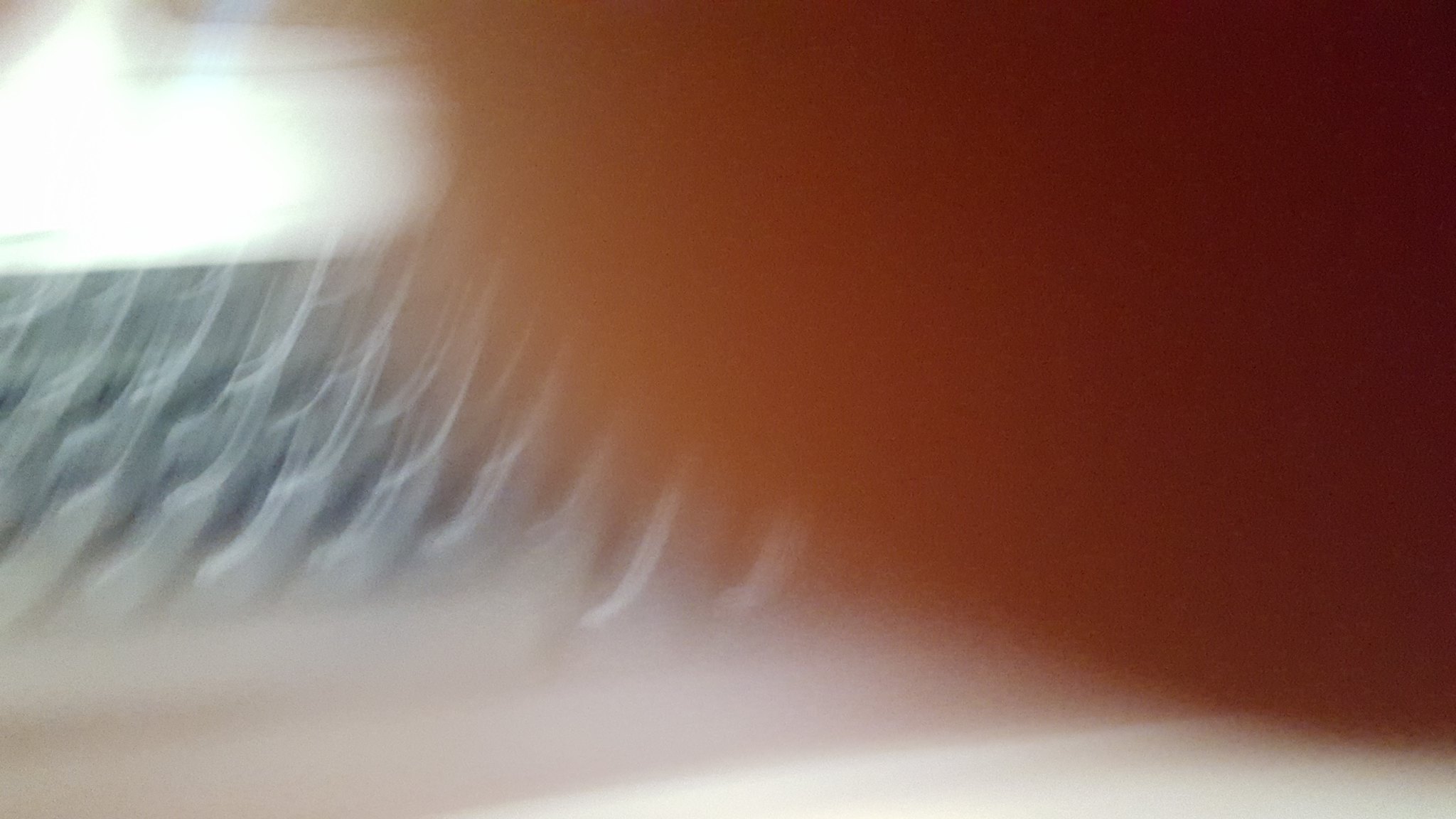This image is a very blurry, low-quality photograph, partially obstructed by a finger placed over the lens from the upper right corner down to the center. The finger, appearing flesh-colored with some shadow, obscures much of the scene. On the right side, it looks like a gray or black keyboard is positioned on a white surface, possibly a shelf or tray desk. A bright light shines above the keyboard, emitting a white glow with a slight green trim. The keyboard, seemingly rectangular, extends from the partially visible area on the left, where motion blur creates elongated, trailing keys that are hard to distinguish. The overall poor focus and obstructions make the details almost indiscernible.